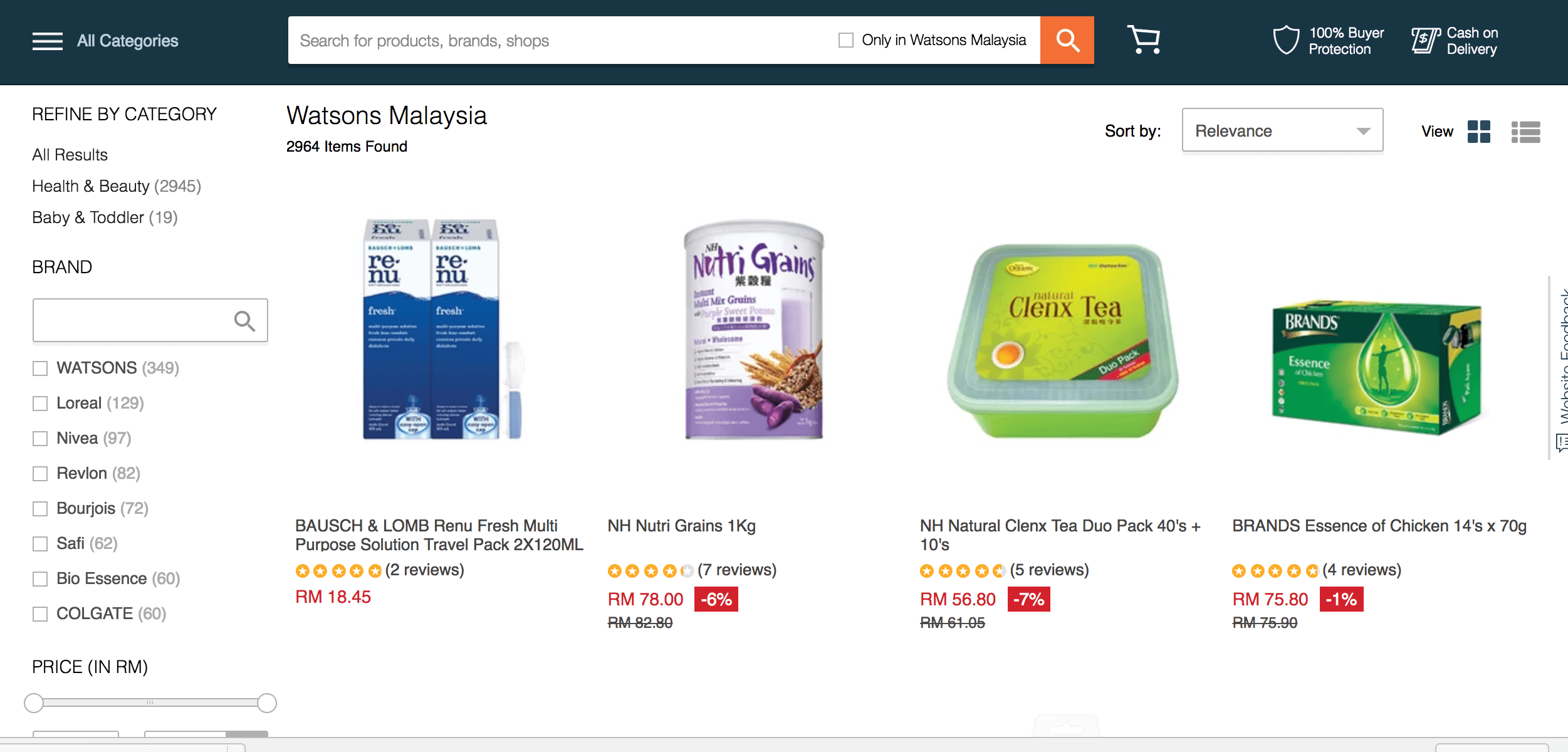This image captures a screenshot of an online shopping page from "Watson's Malaysia," displaying a search result with 2,964 items found. The layout is reminiscent of an Amazon.com page, featuring a search bar at the top for browsing products within various categories. Clearly visible are several product listings, each item accompanied by important details such as brand name, product description, weight, and promotional sales information.

In the center of the image, a product titled "Bausch and Lomb Renew Fresh Multi-Purpose Solution" is prominently featured, suggesting its use for contact lens care. To the right, the website showcases "NH Nutri-Grains" in a 1-kilogram package, followed by "NH Natural Cleanse Tea Dual Pack," which includes 40 plus 10 sachets. Another listed item is "Brand's Essence of Chicken," presented in a 14-pack of 70-gram bottles.

Each product entry includes ratings depicted by stars, pricing information, and any relevant discounts, such as "6% off" or "7% off." These details are conveniently displayed, making it easy for shoppers to compare and choose products.